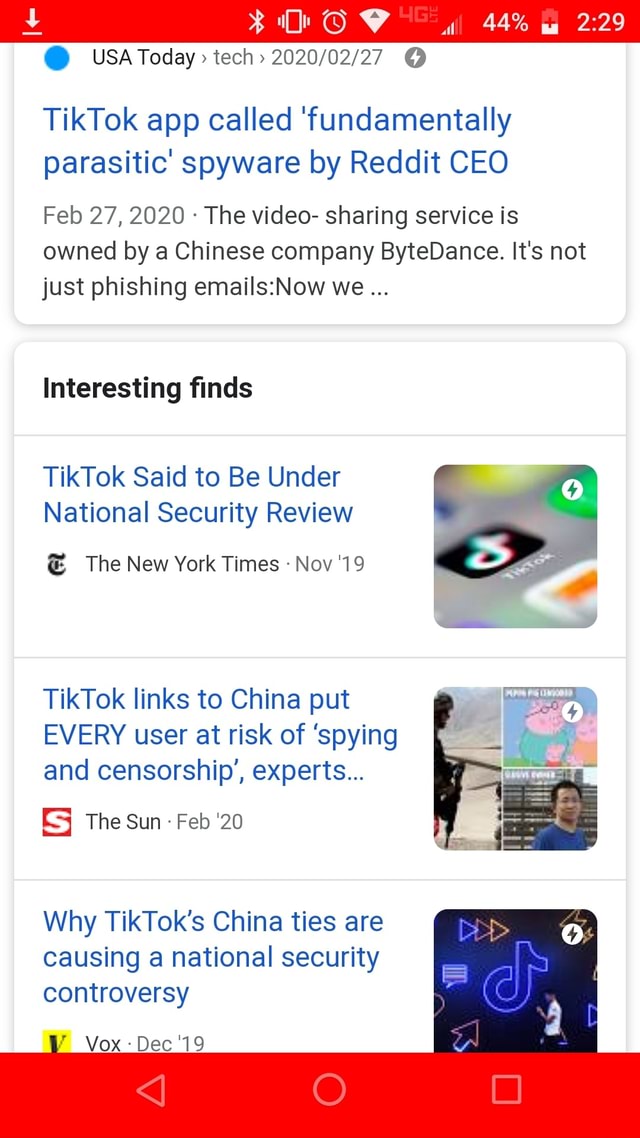This is a screenshot of a news app displayed on a small device, likely a phone. The image shows a red banner at the top, containing various status symbols and notifications, including the time, battery percentage, Wi-Fi connection status, and Bluetooth indication. Below the banner, there is a section titled "USA Today Tech 2020-02-27."

Dominating the screen in larger blue letters is the headline: "TikTok app called Fundamentally Parasitic by Reddit CEO," dated February 27, 2020. Accompanying this headline, a subheader in smaller black text reads: "The video-sharing service is owned by a Chinese company called ByteDance. It's not just phishing emails: now we..."

The interface also features a separate text box headlined in bold black letters: "Interesting Finds." Below this, another section in blue letters informs that "TikTok said to be under national security review," referencing a New York Times article from November 2019.

Further down, yet another text box is present, with the headline "TikTok links to China put every user at risk of spying and censorship, experts..." cited from The Sun on February 20, 2020. Finally, at the bottom of the screen, a small text snippet reads: "Why TikTok's China ties are causing a national security controversy."